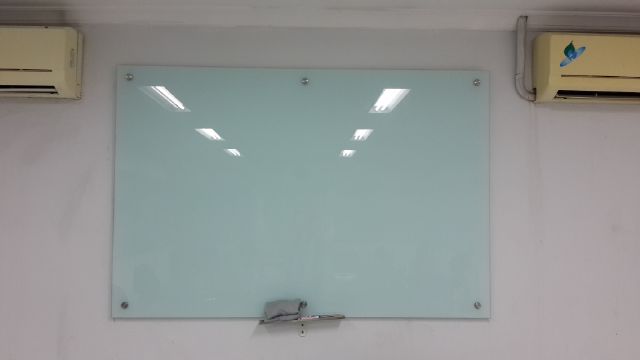The photograph showcases a white or very light gray wall, partially including the white ceiling. Central to the image is a large, highly reflective whiteboard that appears somewhat blueish due to reflections. Affixed to the wall with three silver bolts on the top and two on the bottom, this whiteboard has a small ledge at the bottom center holding a gray cleaning cloth and a pen. Notably, the whiteboard is untouched, with two rows of overhead fluorescent lights and some paper reflected on its surface. High on either side of the whiteboard are yellow or beige air conditioning units with horizontal black openings at the bottom. The unit on the right features a blue butterfly logo or sticker, adding a slight touch of color to the mostly monochromatic setting.